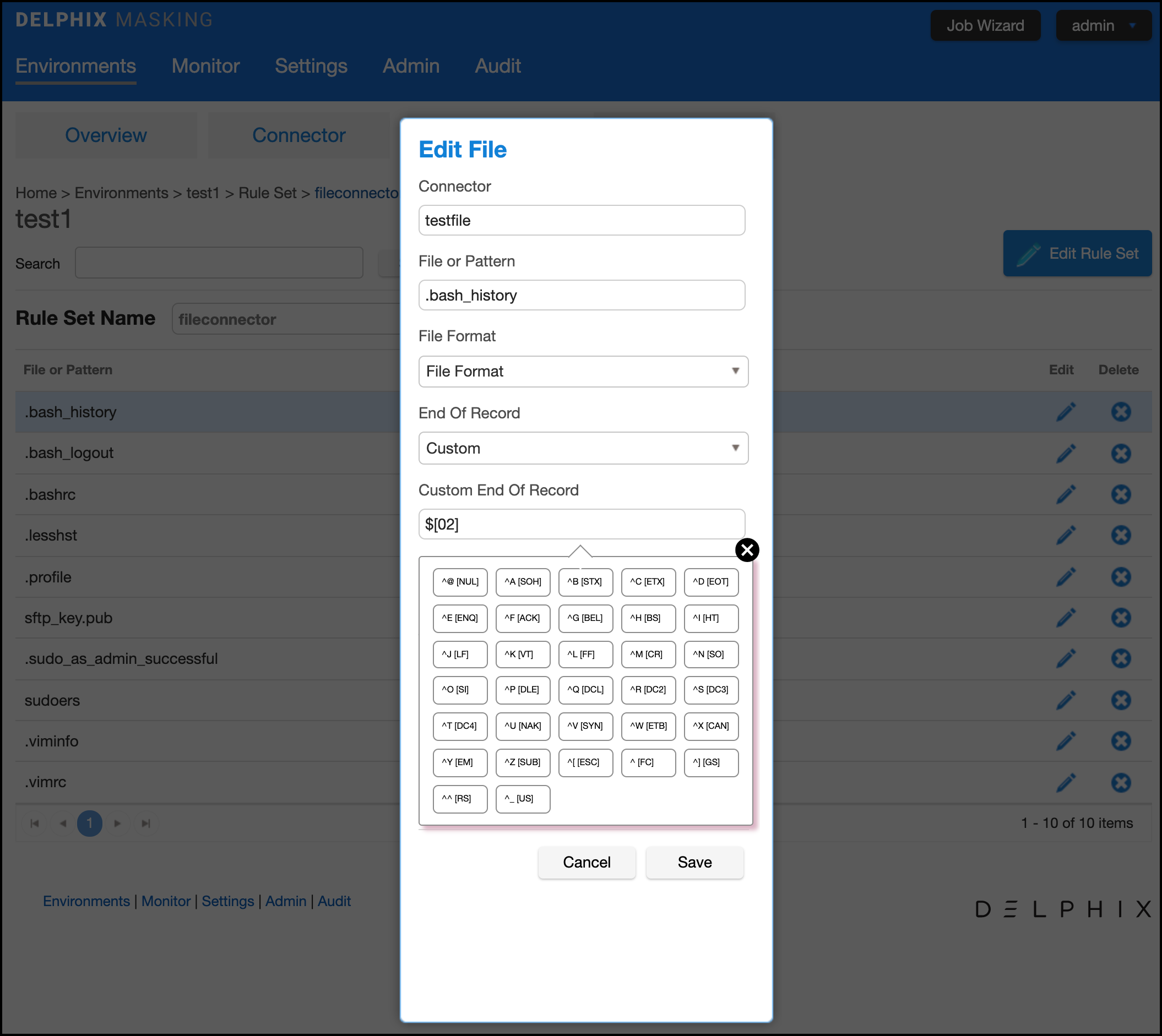The image shows a pop-up overlay from the DELPHIX Masking website, partially obscured by a gray film in the background. The pop-up is a white rectangle that is vertically elongated, with the title "Edit File Connector" prominently displayed in blue at the top. Below the title, there is a data field labeled "Test File or Pattern" where the entry ".bash_history" can be seen under the "File Format" dropdown menu. 

Further down, there is a section labeled "End of Record" with a dropdown menu set to "Custom." This section includes a custom end of record pattern specified as "$[0:end]". Additionally, a dropdown menu extends below this, revealing an array of options organized into a grid of five columns and seven rows. Each button in this grid represents a different selectable option, though the specific chosen option is not immediately clear.

Finally, at the bottom of the pop-up are two buttons: "Cancel" and "Save." Next to the dropdown menu, there is a black circular button with a white "X" for closing the overlay.